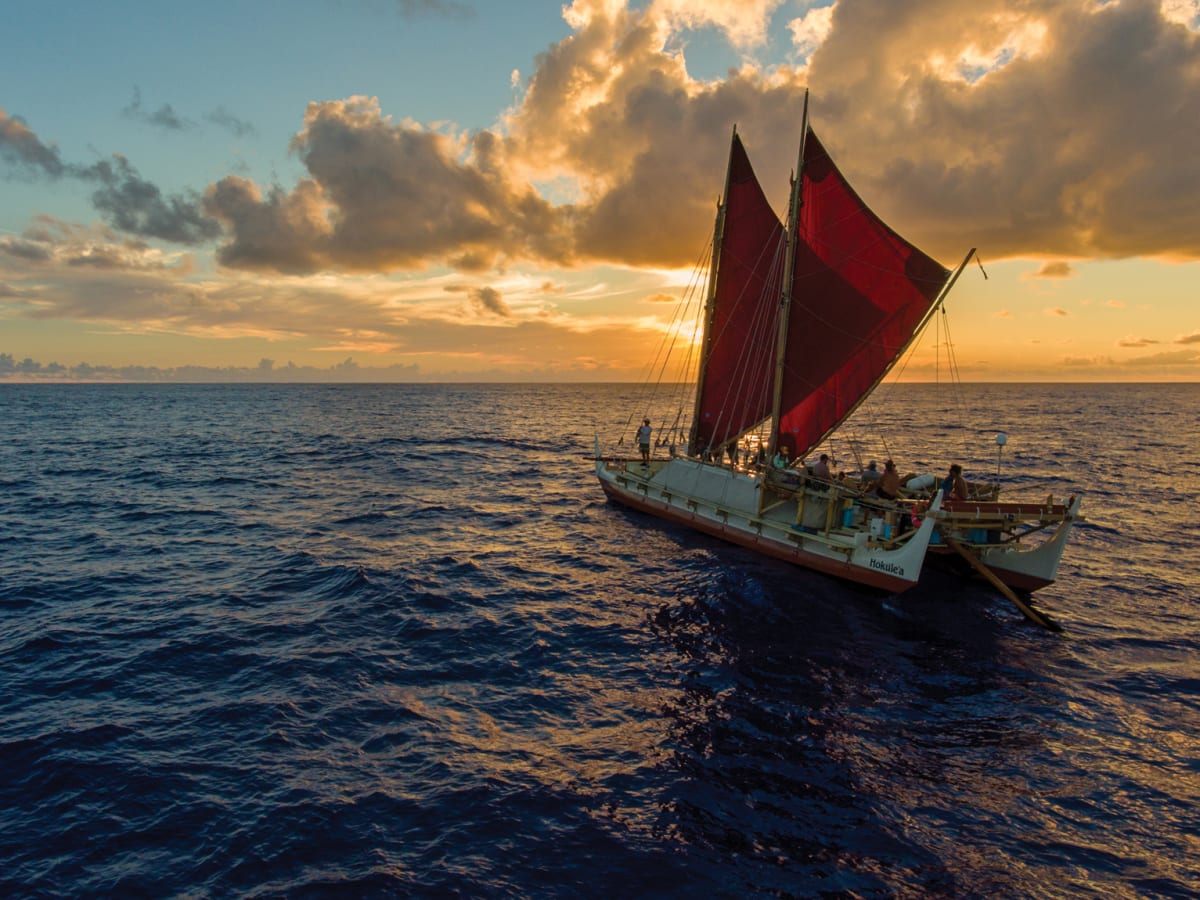The photograph captures a catamaran sailing on a large, dark blue body of water during sunset. The vessel, possibly named Mokulea, features two distinctive triangular red sails connected to a tan-colored mast, with various ropes securing them. The boat has twin floaters and a central platform, which is predominantly white with some wooden elements and a reddish underside. A large wooden oar extending from the back serves as the steering mechanism, partially submerged in the water. The catamaran is populated by what appears to be a mix of around 10-20 tourists, including a figure at the front who may be the captain. The ocean exhibits a calm demeanor with gentle waves, and the sky overhead, a light blue interspersed with dark gray and colorful clouds, sets a picturesque scene as the sun descends on the horizon.